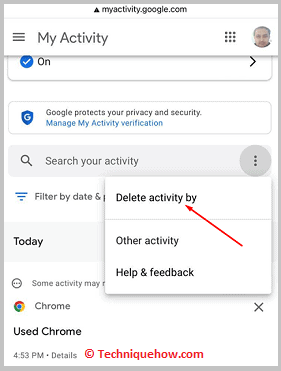The image is a detailed screenshot from the myactivity.google.com page, which is part of Google's suite for managing user data. At the very top, the header clearly displays "My Activity." Just below this, there is a profile icon belonging to the user, featured prominently.

The main part of the screenshot focuses on the "Delete activity by" function, which is both selected and highlighted with a red arrow for emphasis. This dropdown menu allows users to delete their activity data by specific criteria such as date or product type. Additionally, there are other menu options visible, including "Other activity," "Help," and "Feedback."

Highlighted in the screenshot is an example of user activity associated with Google Chrome, demonstrating how one might manage their web browsing history. The bottom of the image includes a watermark from techniquehow.com, emphasizing the source of the guidance.

Overall, the interface provides various tools for users to search, filter, or delete their data across different Google services, potentially including all apps in the Google ecosystem, though this cannot be confirmed with the provided details. The complete layout aids users in efficiently managing their Google account activity.